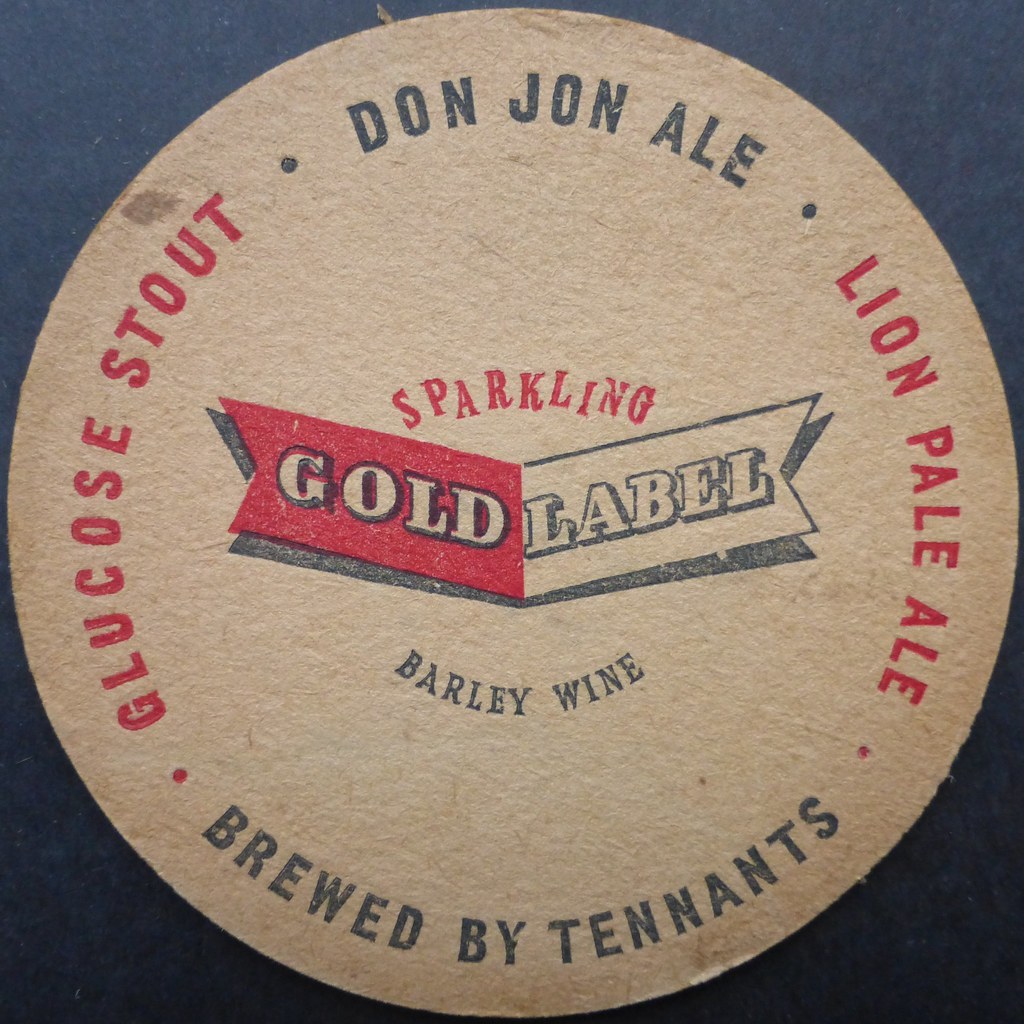This image shows a circular label, possibly a sticker with a somewhat worn and vintage look, on a bluish-black surface. The label itself has a dirty peachy gray background with raised text that gives a 3D appearance. Central to the label are the words "Gold Label" in a distinctive emblem where "Gold" is written in red on a red background on the left side, and "Label" is in white outlined in black on the right side. Above this emblem, the word "Sparkling" is prominent in red text, and below it, "Barley Wine" appears in black.

Encircling this emblem are multiple inscriptions: "Don John Ale" at the top in gray, "Glucose Stout" to the left in red, "Lion Pale Ale" to the right in red, and "Brewed by Tenants" at the bottom in gray. The label gives an impression of an old sticker, with smudge spots and a rough texture, evocative of a barley wine sticker, affirming its rich heritage.